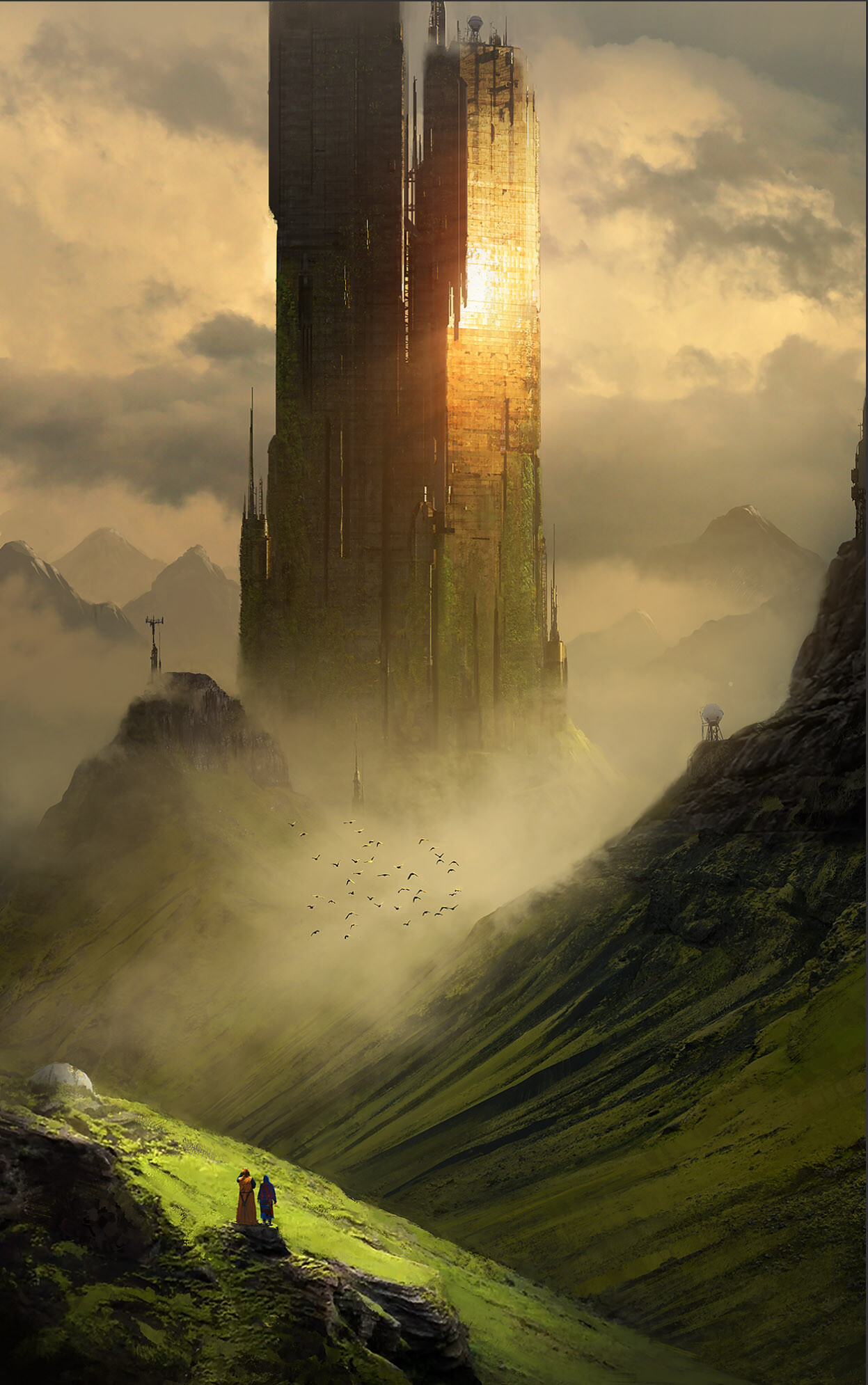This vertical rectangular image, likely a digital painting, captures a striking science fiction scene. Dominating the center is a monumental, man-made rock formation with two towering structures, one extending out of the image's upper edge. The formation, primarily brown with orange highlights, exudes a shimmering golden hue as light reflects off its surface. The structure features smooth surfaces interspersed with broken, jagged edges and a central seam, suggesting a futuristic, possibly abandoned skyscraper with glistening yellow walls and glass windows. Dark, ominous clouds loom in the background, casting a hazy, smoke-laden sky. 

In the foreground, the emphasized vibrant green landscape slopes dramatically, adorned with lush, moss-like grass that almost appears real. This greenery extends up the side of another rocky outcrop, creating a dynamic valley scene with gray rock formations. Two small figures stand on a rock precipice in the lower left corner, seemingly gazing up at the towering structure. Adding to the depth, a flock of birds navigates through the fog and clouds, accentuating the image's ethereal and mysterious atmosphere.